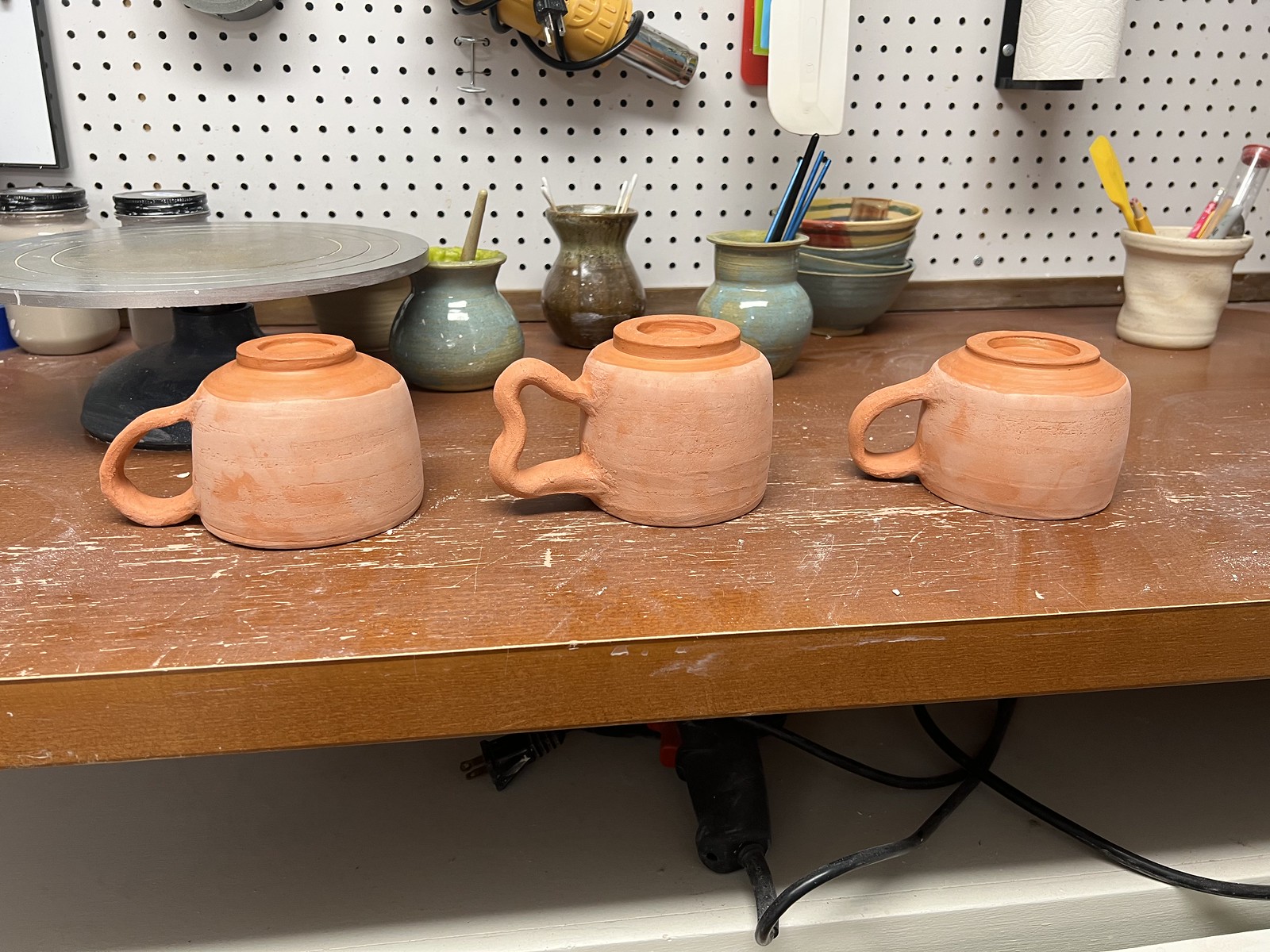The image depicts a detailed scene of an active potter's workbench. The wooden bench, visibly worn with scratches and scars, sits atop a lower white bench. Between these two surfaces, power tools and electrical cords are partially visible. The main workbench holds three upside-down, unfired terracotta mugs, identifiable by their handles. A small pottery wheel is situated to the left. In the background, a variety of finished, glazed pottery pieces are present, many repurposed to hold utensils like pencils, paintbrushes, and other pointy tools. Notably, a raised platter with a gray marble surface stands about eight inches off the tabletop. Additionally, there’s a slightly misshapen beige bowl filled with potter's tools, and several glass jars containing a white substance. A pegboard behind the bench displays various mounted tools, a heat gun with its cord looped around it, and a roll of paper towels. Some items on the pegboard are cut off from the picture, limiting their visibility.